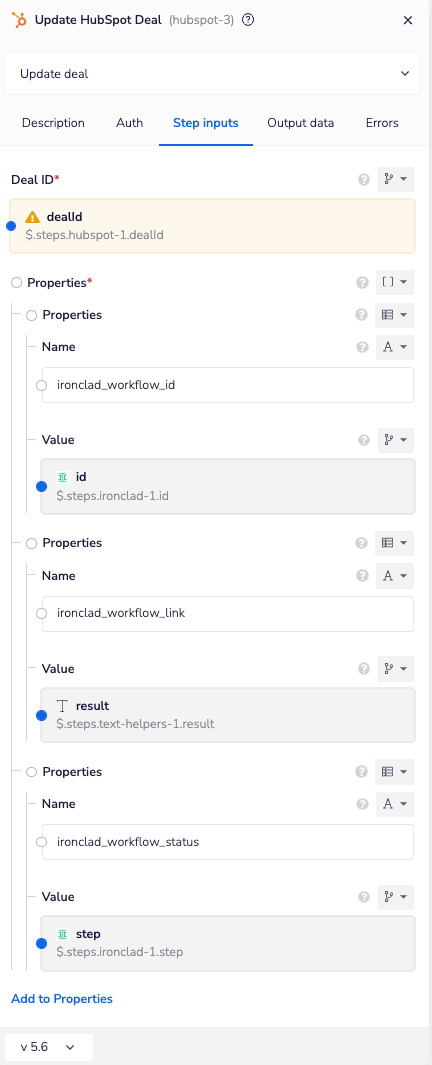This image is a detailed screenshot, likely captured from a cell phone given its portrait orientation. The main area of the screenshot features a predominantly white background, with a gray rectangle positioned along the top edge. In the upper left corner of this gray bar, there is an orange logo that appears to be associated with a company or function named "Update."

At the top of the interface, the header reads "Update HubSpot Deal (HubSpot 3)." Directly below the header, there is a white drop-down menu currently displaying the option "Update Deal." 

A row of tabs is lined up beneath the drop-down menu, labeled as follows: Description, Auth, Step Inputs, Output Data, and Errors. The tab titled "Step Inputs" is highlighted in blue and underlined, indicating it is currently selected.

Under the "Step Inputs" tab, there is a field labeled "Deal ID" marked with a red asterisk, indicating it is a required field. A yellow rectangle surrounds this field, accompanied by a caution symbol and the text "Deal ID," signifying an error or alert message.

Below this, various technical fields are displayed, each identified as "Property" and "Value." These fields are accompanied by drop-down menus filled with different symbols, suggesting the presence of multiple options for each technical attribute. This setup suggests the interface is designed for a technical task, potentially related to computer programming or web design within the HubSpot ecosystem.